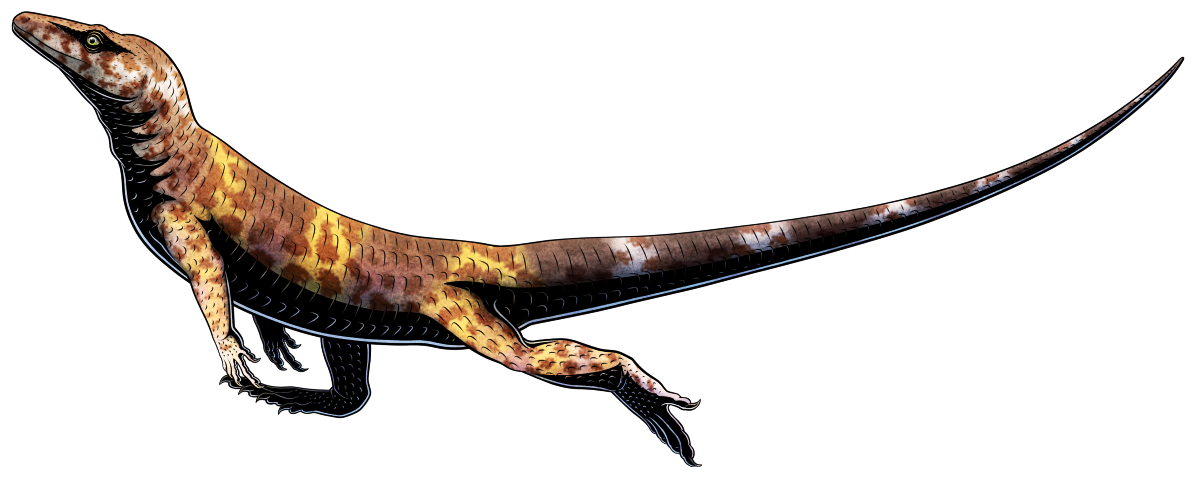The image depicts an artistic rendering of a gecko-like creature, seen from a side view, against a pure white background. The gecko is facing left, with its long, tapering tail extending to the right. Its body displays a colorful pattern, with dark brown as the base color, interspersed with patches of yellow and white. Notably, the tail is darker brown with white specks and tapers off towards the tip.

The gecko appears to be mid-motion, giving an impression of walking or running. Its right hind leg is in shadow and flat on the ground, while the left hind leg has only its toes touching the ground, as if in stride. The front legs are smaller and hang by its sides. The back legs are longer, with more pronounced toes, including a thumb-like toe with claws.

The head of the gecko, which resembles that of a lizard or small dinosaur, is light brown with darker spots and a rounded front snout akin to a crocodile. The eyes are small, yellow, with dark pupils and are surrounded by dark areas. The overall composition and color scheme give a detailed and lively appearance to the creature, making it appear as if it is in motion on a blank canvas.